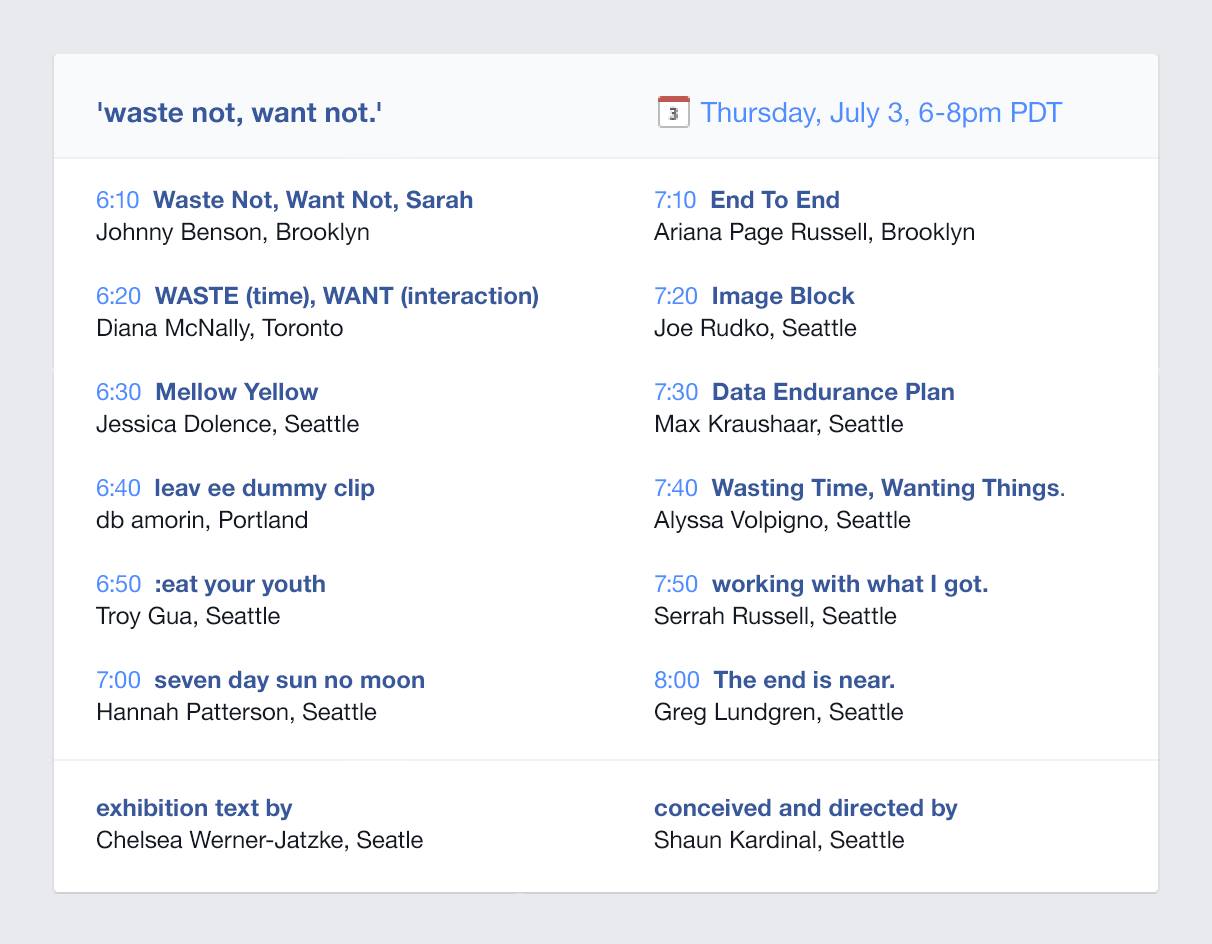This image is an event schedule presented on a mellow yellow background. The schedule appears to be organized around a central theme, "Waste Not, Want Not," displayed in dark blue text at the top left within single quotation marks and lowercase letters. Specific events are outlined as follows:

- **6:10 PM:** "Waste Not, Want Not" by Sarah and Johnny Benson, Brooklyn.
- **6:20 PM:** "Waste Time, Want Interaction" by Diana McNally, Toronto.
- **6:30 PM:** "Mellow Yellow" by Jessica Dolan, Seattle (with no additional details provided).
- **6:40 PM:** "Lee E Dummy Clip" by DBMR in Portland, using a slightly lighter blue for the time.
- **6:50 PM:** "Here Youth Choi Gloss" by an individual from Seattle.
- **7:00 PM:** "Seven Days, Seven Nights" by Hannah Patterson, Seattle.
- **7:10 PM:** "I Ran a Page for Us" by someone from Brooklyn.
- **7:20 PM:** "Image Brought Up to the Root Cause" by an individual from Seattle.
- **7:30 PM:** "Data Endurance Plan" by Max Carousel, Seattle.
- **7:40 PM:** "Wasting Time, Wanting Things" by Alistair Wild, Seattle.

The event is scheduled for Thursday, July 3rd, from 6:00 to 8:00 PM PDT, as indicated at the top right of the event image.